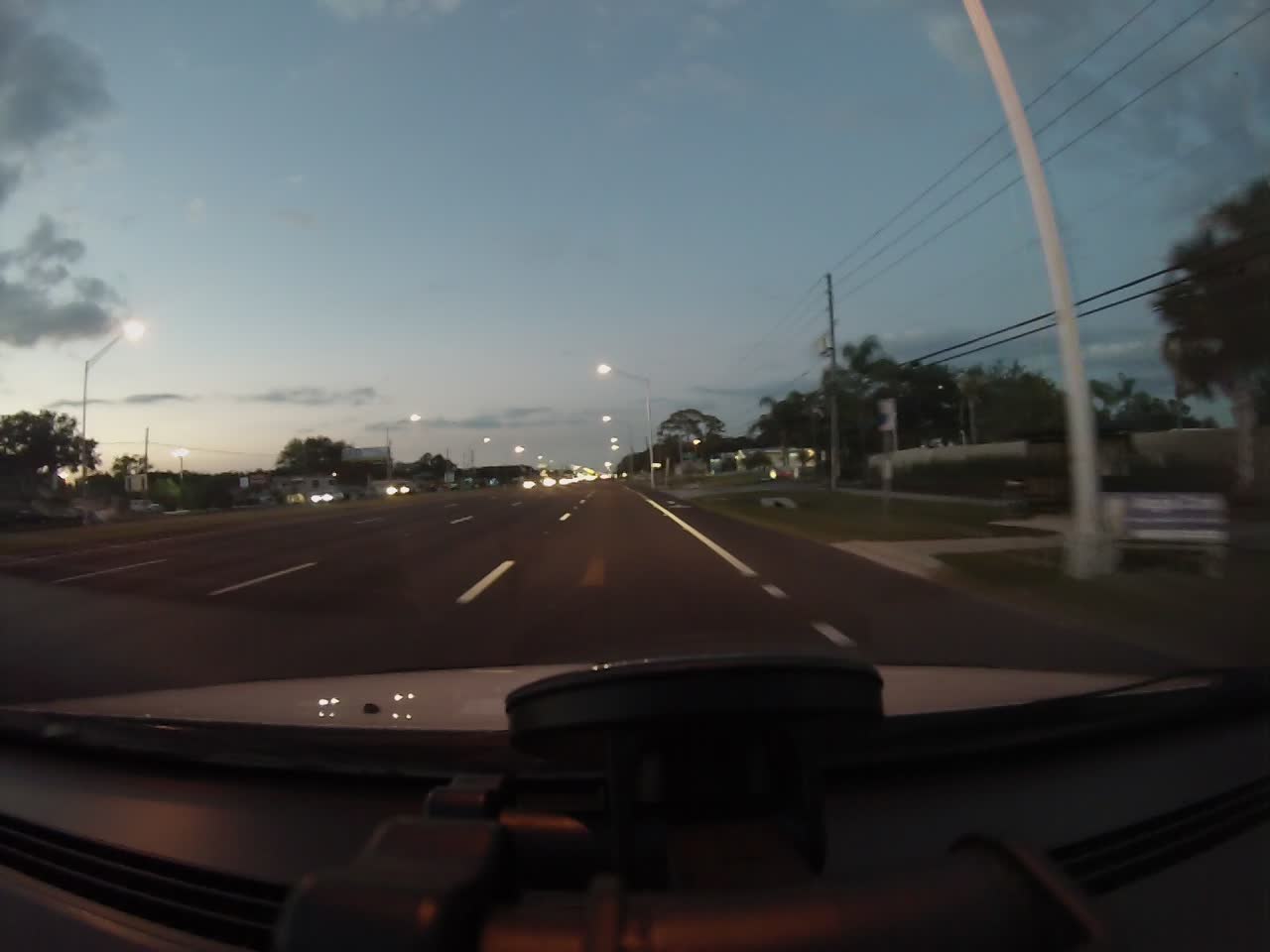This photograph offers a view from behind the windshield of a car traveling down a four-lane highway. Taken during dawn or dusk, the sky is faintly illuminated while the headlights of vehicles pierce through the dim light. The highway, bustling with oncoming traffic on the opposite side, features a grassy verge and a sidewalk to the right. Streetlights and posts dot the roadside, casting faint glows. Low-lying buildings, possibly residential homes or small businesses, are visible beyond the grassy area. The image, slightly blurred and of lower resolution, shows the top edge of the car's dashboard, emphasizing the in-motion perspective of this early morning or late evening commute.